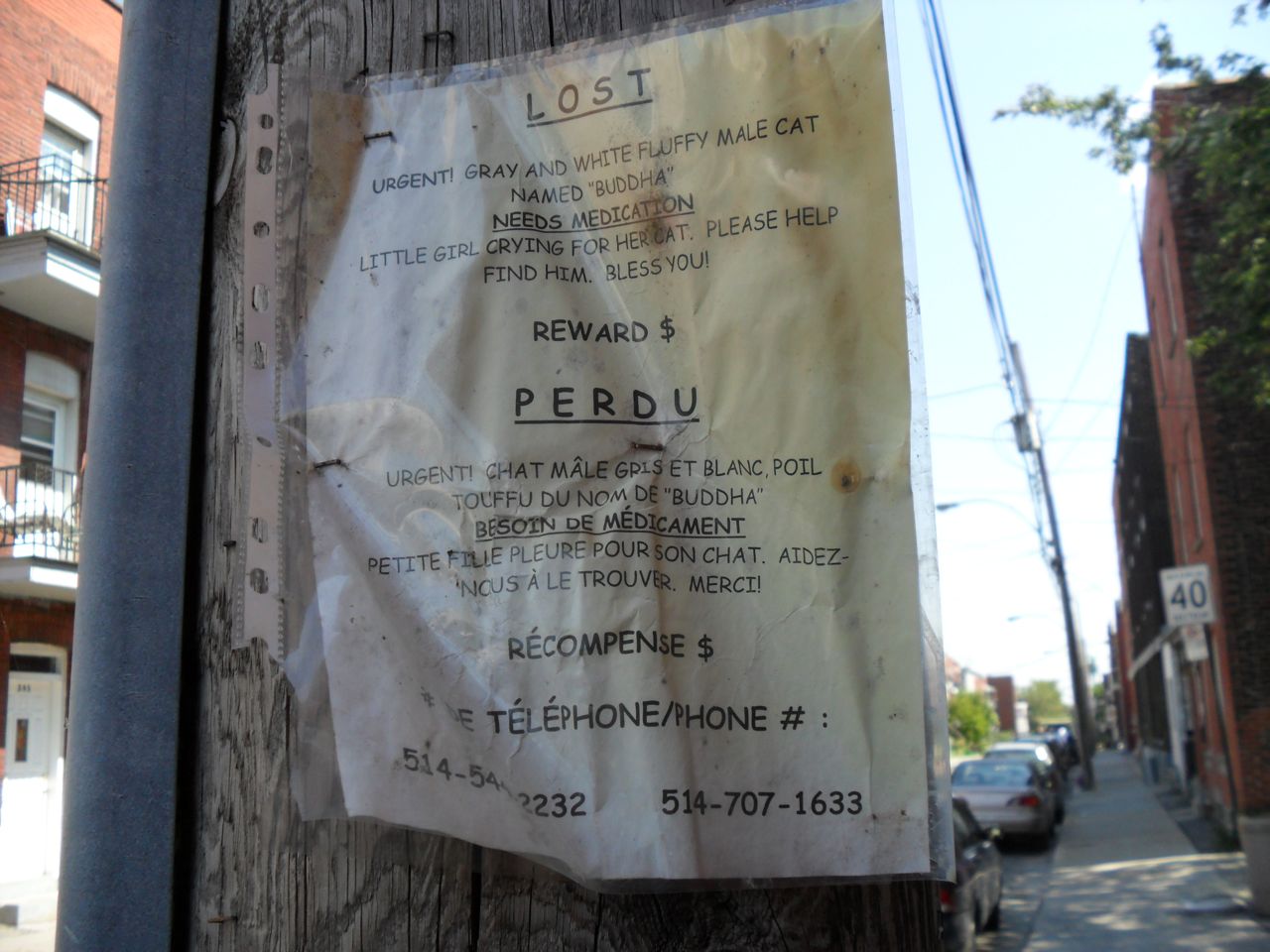In an urban neighborhood, possibly in Canada given the bilingual signage, there is a tall red brick apartment building complex visible across the street, suggesting an older, potentially gentrified area. The scene features several other red brick buildings, parked cars, and patches of greenery. Dominating the image is a lighter-colored wooden telephone pole, central to the composition. Affixed to the pole is a noticeably weathered, laminated sign. The paper within, creased and yellowing from exposure to the elements, prominently displays an urgent plea in black letters: "LOST. Urgent. Gray and white fluffy male cat named Buddha. Needs medication. Little girl crying for her cat. Please help find him. Bless you. Reward $." Below the English text, the message is repeated in French, emphasizing the urgency and locality, with the contact information at the bottom. The detail and dual language suggest a community-oriented effort to find the missing pet.